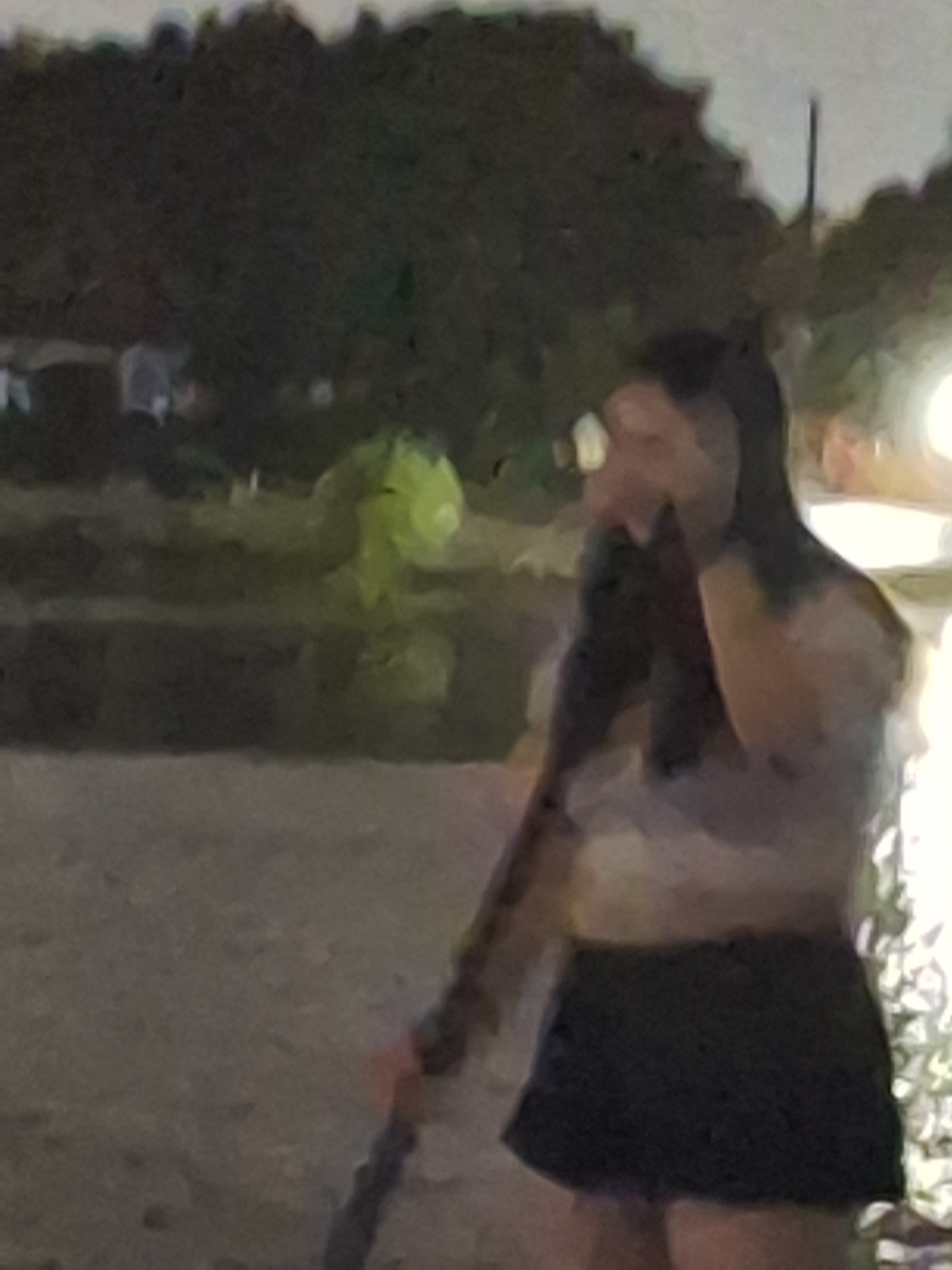The image depicts a heavily pixelated or blurred scene, resembling a poorly filtered or abstract painting. In the foreground, slightly to the right, stands a young pale-skinned woman with long, dark (possibly black or brown) hair. She is dressed in black shorts and a white top with hints of purple. Her left arm is bent at the elbow, with her hand near her face, possibly wearing a black watch on her wrist. In her right hand, she appears to be holding a long object that could be an oar, stick, or bat.

The background features a body of water that looks reflective, indicating light shining off its surface, and is dark gray or black in color. Near the water's edge are trees and possibly some buildings or houses with a fence. Part of a large pole is also visible. On the upper part of the image, the sky is an ominous dark gray, further casting a shadowy ambiance over the scene. The overall image has an appearance reminiscent of fragmented plastic, lacking clear details and giving a surreal, stained-glass effect.